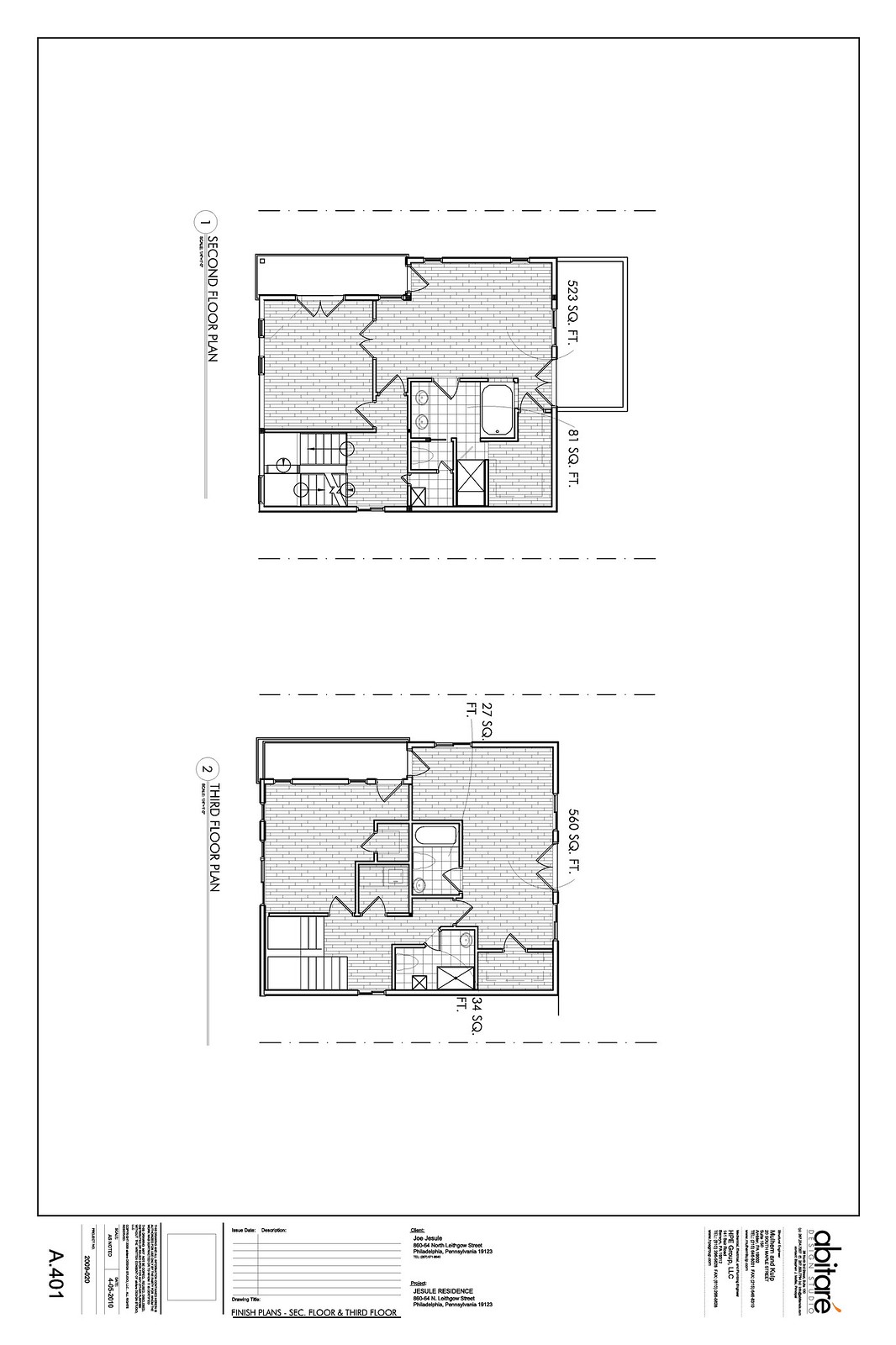In the detailed floor plan shown, the layout is divided into distinct sections with specific measurements and features. Starting from the top left, there is a large rectangle indicating a spacious area. To the bottom left, there are stairs depicted with several circular symbols on them. 

Moving to the middle section, we find a swinging doorway leading to a bathroom equipped with two sinks, a bathtub, and another door leading to a toilet area. Adjacent to this bathroom, there is a square with a cross through it, possibly representing an additional functional area or utility space.

On the right side, there are several foreplanes. The first foreplane mentioned at the bottom right has an annotation that reads "I'll be better..." and covers an area of 523 square feet. Above it, the second foreplane is visible, while the third foreplane is located at the bottom of the illustration, measuring 560 square feet.

The bottom section includes another bathroom with a notation of 81 square feet. This area includes a toilet, sink, and bathtub. There is an entryway marked by a square, with doors swinging into it on the left side.

Overall, this floor plan displays a meticulously detailed layout, featuring multiple rooms, bathrooms, a large open area, and an entryway with accessible stairs.